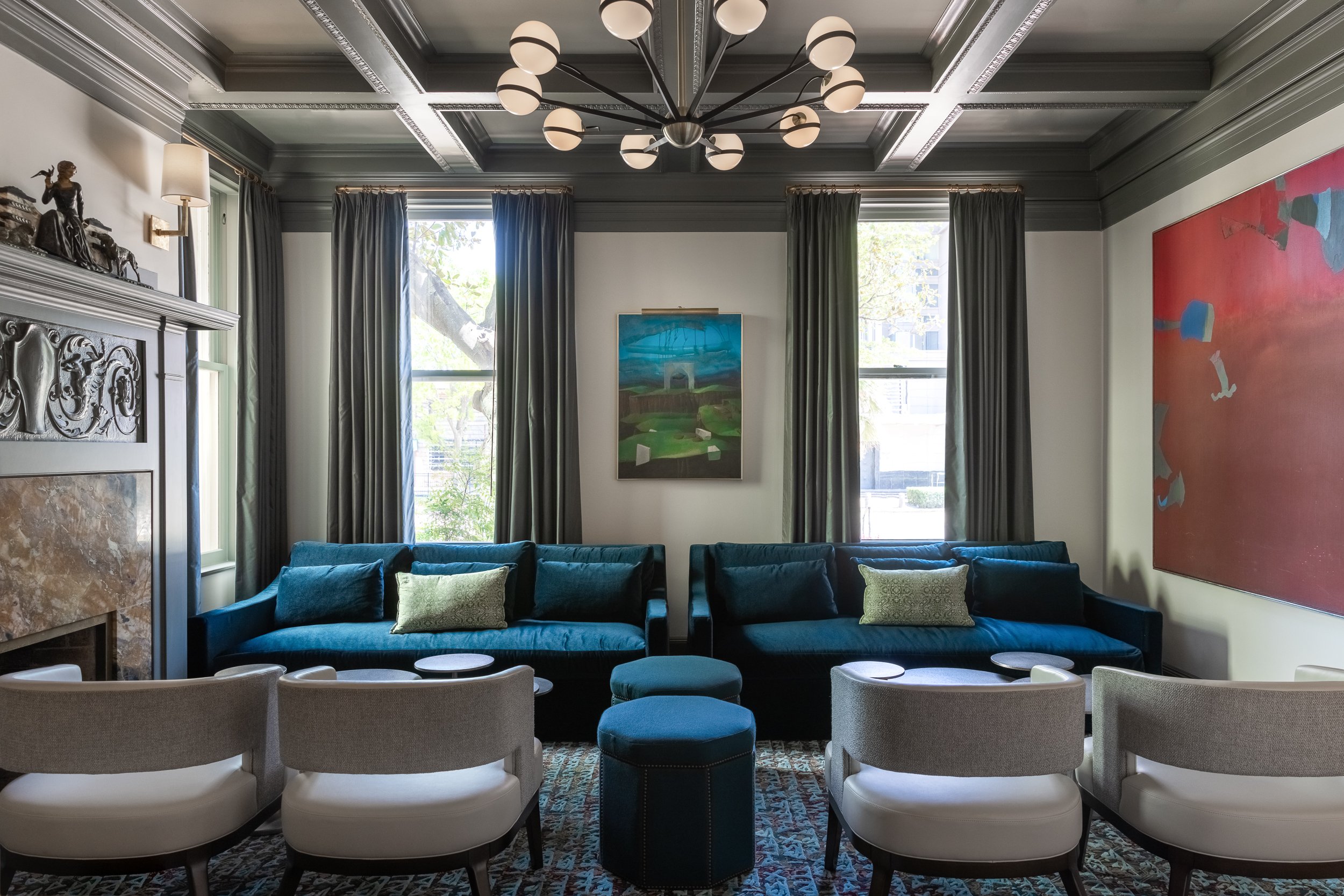The image portrays an elegantly furnished sitting room, illuminated by both natural and artificial light. Dominating the back wall are two tall, open windows with light streaming through, flanked by long, gray curtains. Between the windows, a blue-and-green conceptual painting with an indistinct subject adds a touch of color. Below the windows, two identical blue sofas are arranged side by side, each adorned with blue cushions and a single white throw pillow. Blue upholstered ottomans are positioned in front of the sofas.

The room features four white upholstered chairs, with two on the right and two on the left, facing the sofas. These chairs are aligned in a row, with their backs to the viewer. Between the seating arrangements are small wooden tables and two more blue upholstered tables, possibly ottomans or footstools.

On the right wall hangs a striking piece of conceptual art primarily rendered in red with splashes of blue. The left side showcases an ornate marble fireplace, topped by a statue, likely of a woman, resting on an elaborate mantle. Above the fireplace is a lighting sconce.

The ceiling of the room is intricately designed with rectangular sections and is adorned with a modern, silver globe chandelier. The chandelier features black spokes with globe lights at their ends, reminiscent of a solar system. The floor features a richly colored carpet, interwoven with blue and red hues, complementing the room’s overall palette.